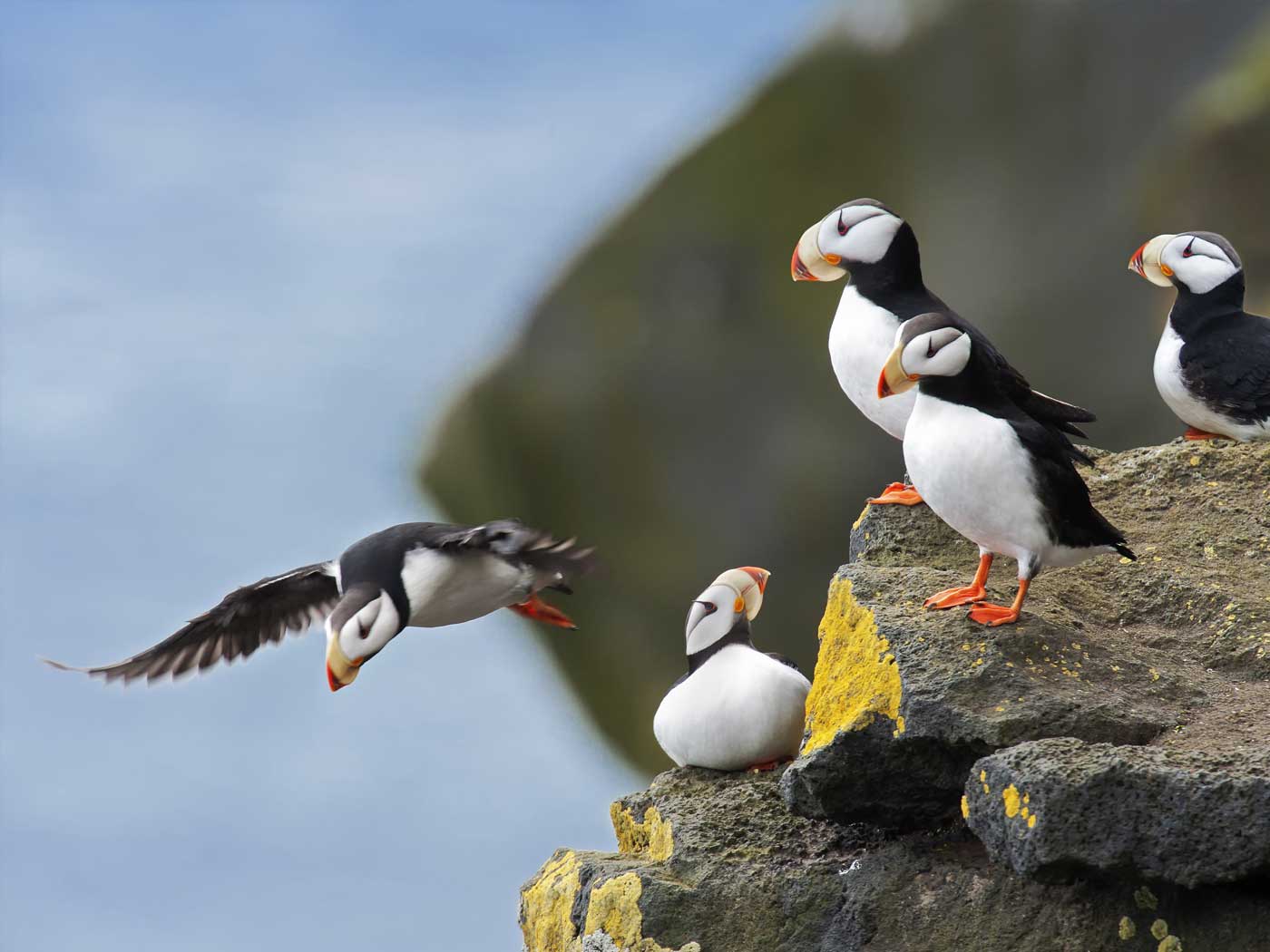This is a detailed photograph capturing five vibrant puffins near the edge of a cliff, with a blurred background that hint at a nearby body of water. The puffins, with their distinctive black backs, white chests, and vivid yellow beaks tipped with orange, are perched on large slabs of rock covered in yellow moss or lichen. One puffin has just leapt into the air, wings extended, and is flying down towards the bottom left. The remaining four puffins are either standing or sitting on the right-hand side rocks. Three puffins are positioned higher on an outcropping, all gazing towards the left, while the fourth puffin, perched lower on another rock, looks up and to the right at the other puffins. The scene is framed by the striking yellow-edged rocks and the puffins' bright orange feet, creating a vivid contrast against the blurred backdrop that merges seamlessly into what appears to be water and sky.